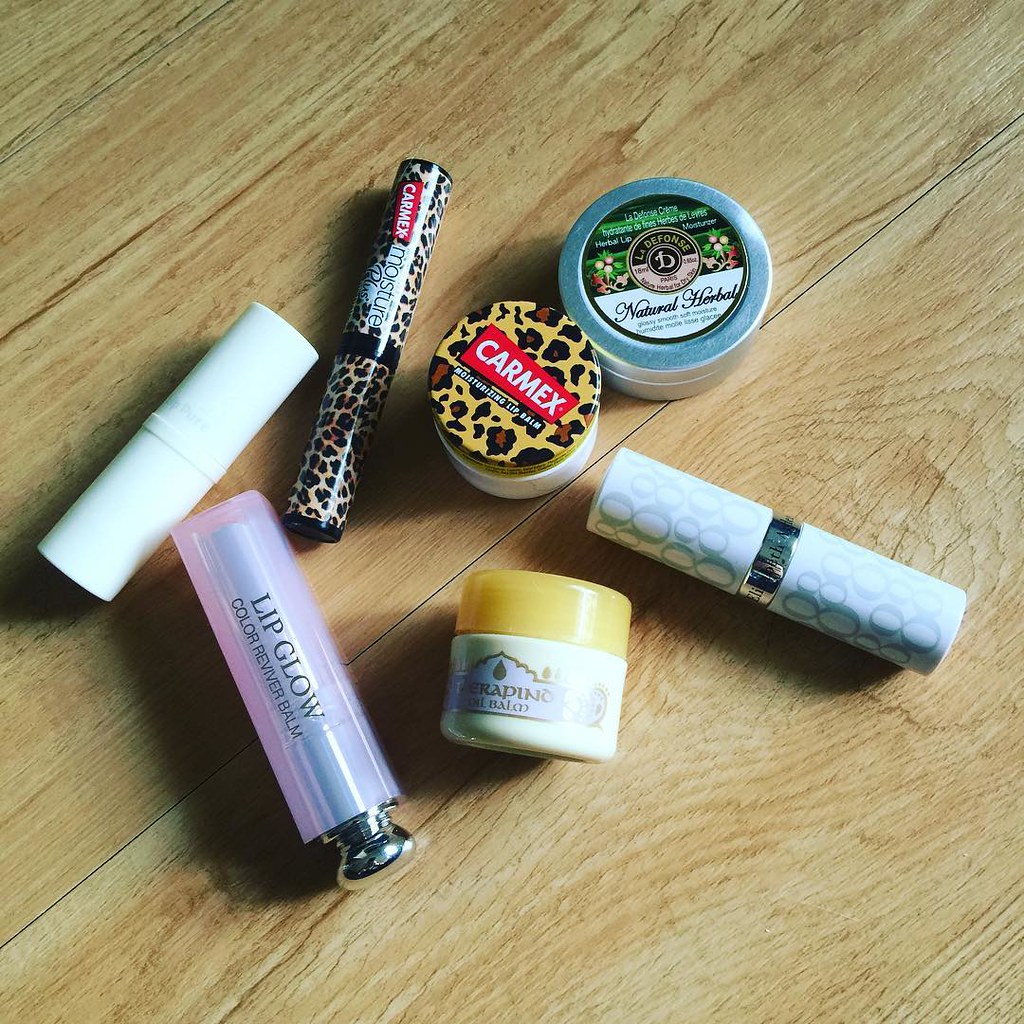In the image, there are seven different chapsticks displayed on a beige, wooden table. Three of the chapsticks are in round containers that you open by removing the top and apply using your finger. The remaining four chapsticks are in stick form, designed to be rolled directly onto the lips. Two of the chapsticks feature a cheetah print design; one of these also has the brand name "Carmex" on it. Another chapstick is labeled "Lip Glow Color Reviver Balm" and is of a pinkish hue. There is also an all-white chapstick, and another one that is blue with a pattern of "O"s on it. Additionally, one of the chapsticks is noted to have "Natural Herbal" on its label.